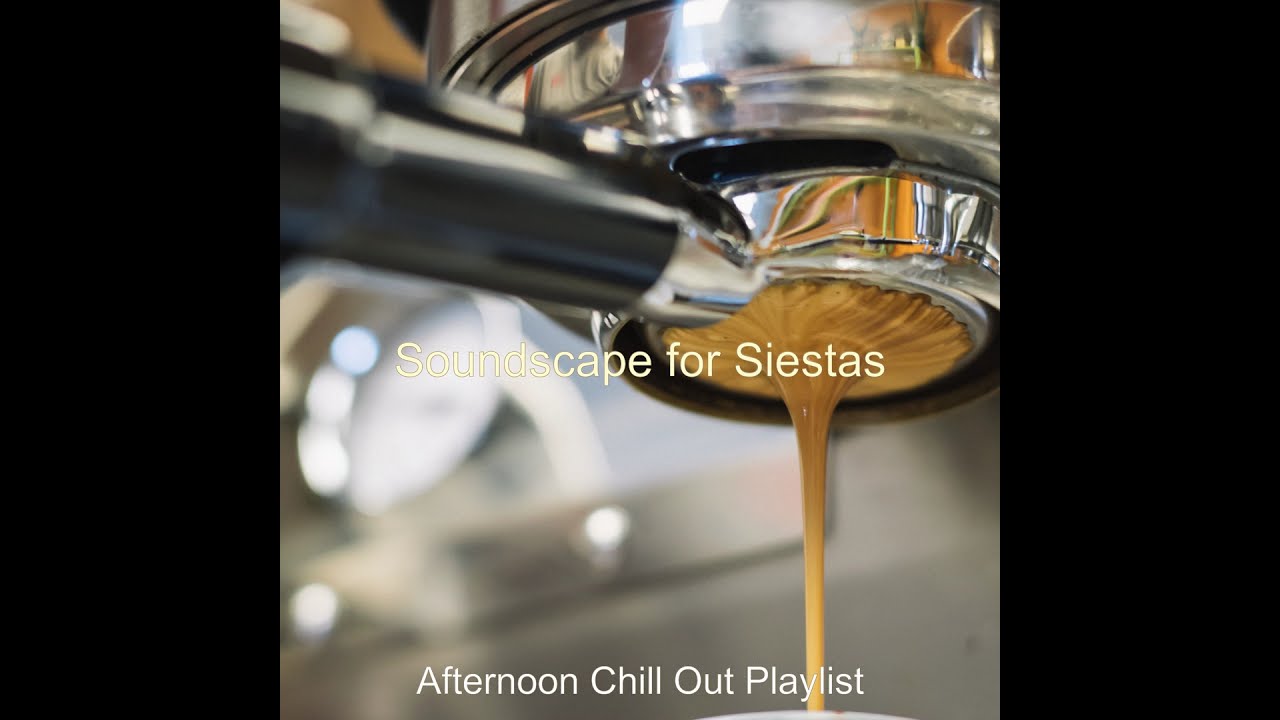This image is a color, square-format photograph inset into a horizontal landscape layout with black vertical strips on either side. It features a detailed close-up of an espresso machine, capturing the moment as rich, brown espresso flows continuously from the filter at the bottom of the device. The espresso machine has a circular component with a black handle and metal parts. The background reveals more metallic elements, emphasizing the industrial design of the coffee maker. Across the center of the photograph, white text reads "Soundscape for Siestas," and at the bottom, it also states "Afternoon Chill Out Playlist." This image might serve as a promotional cover for a music playlist or album, focusing on a theme of relaxation and leisure, enhanced by the photorealistic and representational style of the artwork.